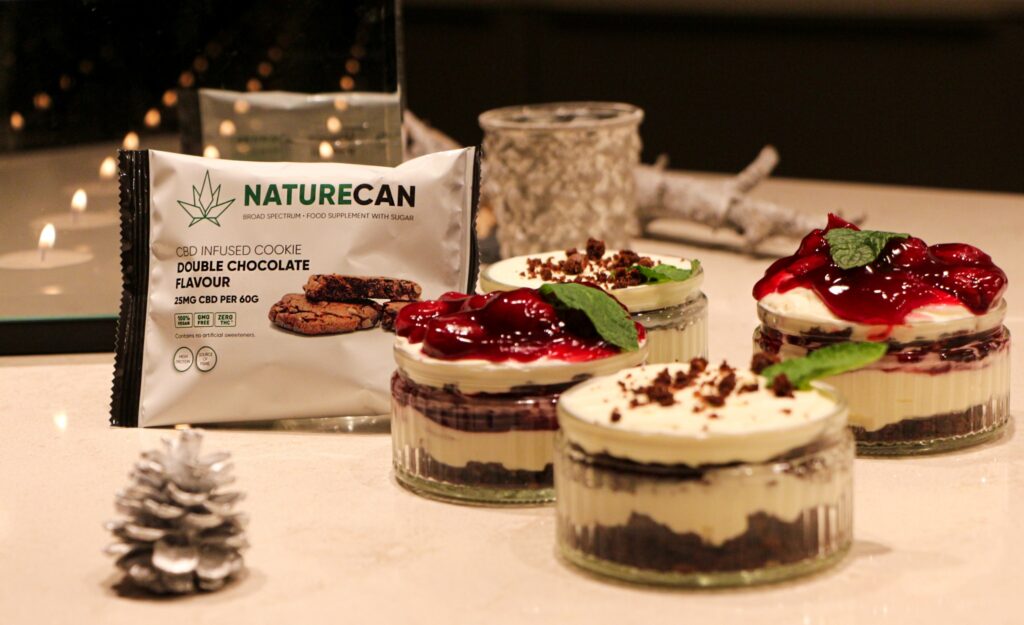This image features a pristine white table set with four meticulously layered desserts, each presented in small, round glass bowls. The desserts are positioned toward the center and center-right of the frame. Each dessert layers a chocolate cookie base alternated with white cream, topped with either cookie crumbles or strawberry puree. To the left of the desserts, a white package captures attention, advertising "Nature Can" CBD-infused double chocolate cookies, featuring a detailed label including "25 milligrams CBD per 60 grams." A white-painted pine cone and a small white stick adorn the table, enhancing the wintry, serene atmosphere. The background, predominantly dark, includes a glass surface that reflects the package and a faint candlelight, contributing to an elegant and cozy setting.